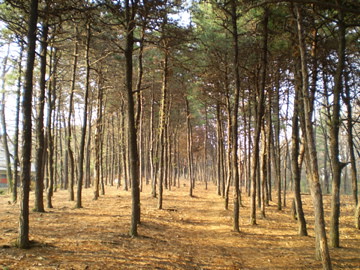The photograph depicts a meticulously maintained forest area with numerous very tall trees characterized by their thin trunks and dense green foliage at the top. The forest floor is strikingly clear of any vegetation, displaying a sandy, yellowish hue with no grass or other ground cover. The trees are arranged professionally and appear to be managed, possibly for purposes such as fire prevention or future use in a paper mill or power plant. Light blue sky can be glimpsed through the dense canopy of leaves, hinting at the open, airy feeling above. To the left side of the image, there is a hint of a building-like structure, adding a touch of human presence to the natural setting. The overall impression is one of a clean, well-organized forest, possibly part of a park or a designated forestry area.